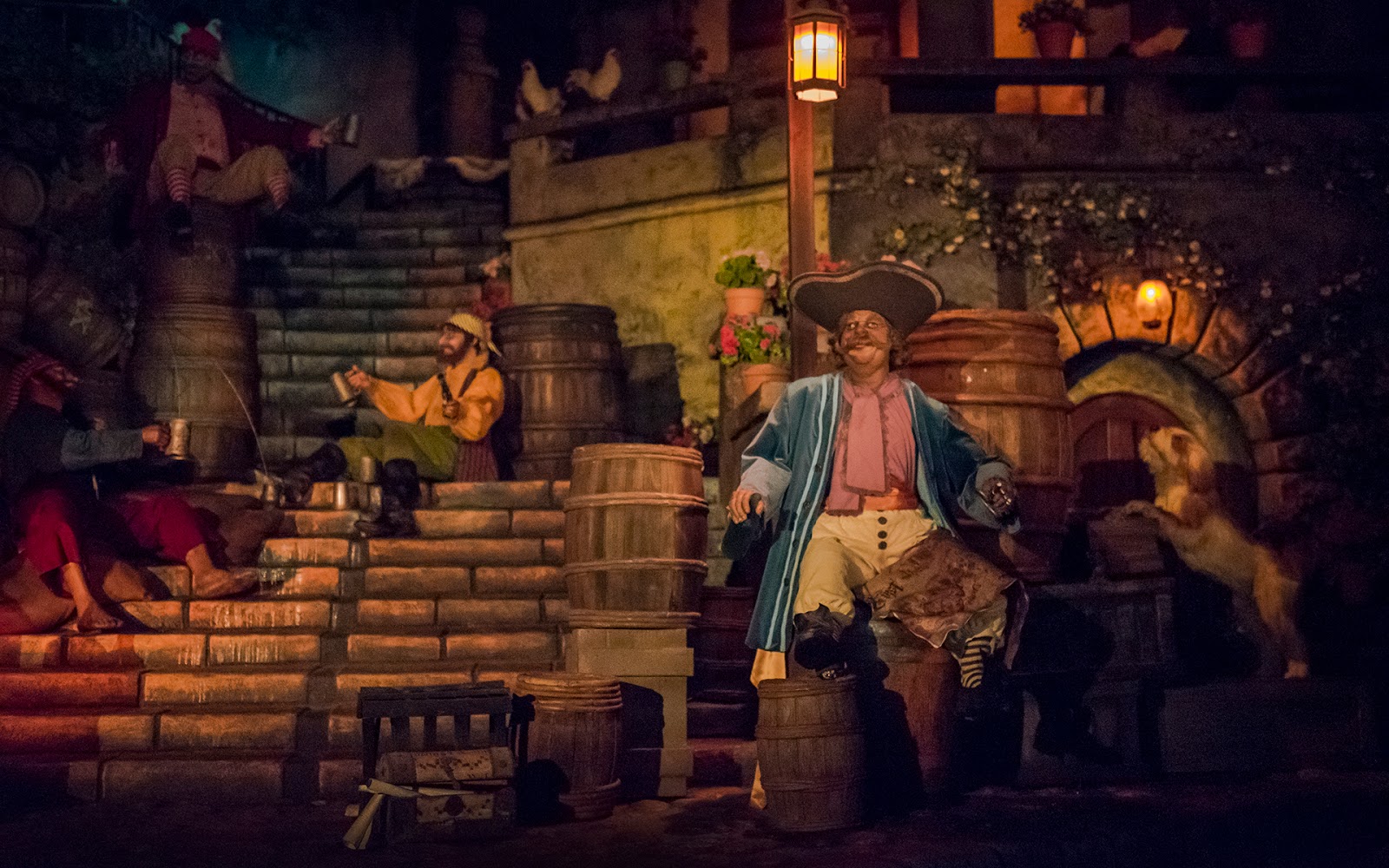The scene is a richly detailed painting or drawing reminiscent of an old Disneyland attraction, specifically the Pirates of the Caribbean. The setting features a lively and bustling street with a set of steps ascending from the foreground into the background. These steps seem to lead to a bar or similar establishment. Several pirates populate the scene; one is seated in the middle of the steps, leaning against a barrel and holding a mug which could be filled with beer or gin. Another pirate, dressed in a pink shirt and blue coat with a pirate hat, is prominently in the foreground, accompanied by a dog standing on its hind legs next to a barrel. This pirate appears to have a wooden peg for a leg, and another one in the group has a hook for a hand.

The steps are decorated with barrels, some of which appear to be leaking, and there are planters in the background with pink and white flowers. A lamppost and vines growing on a nearby building add to the intricate setting. Additionally, there is a treasure chest at the base of the stairs and wooden cages, possibly for the chickens that are perched on a railing towards the top of the building. The overall ambiance of the scene evokes the rustic and adventurous spirit of pirate life, with detailed attention to period-specific attire and accessories like pirate hats and beards.